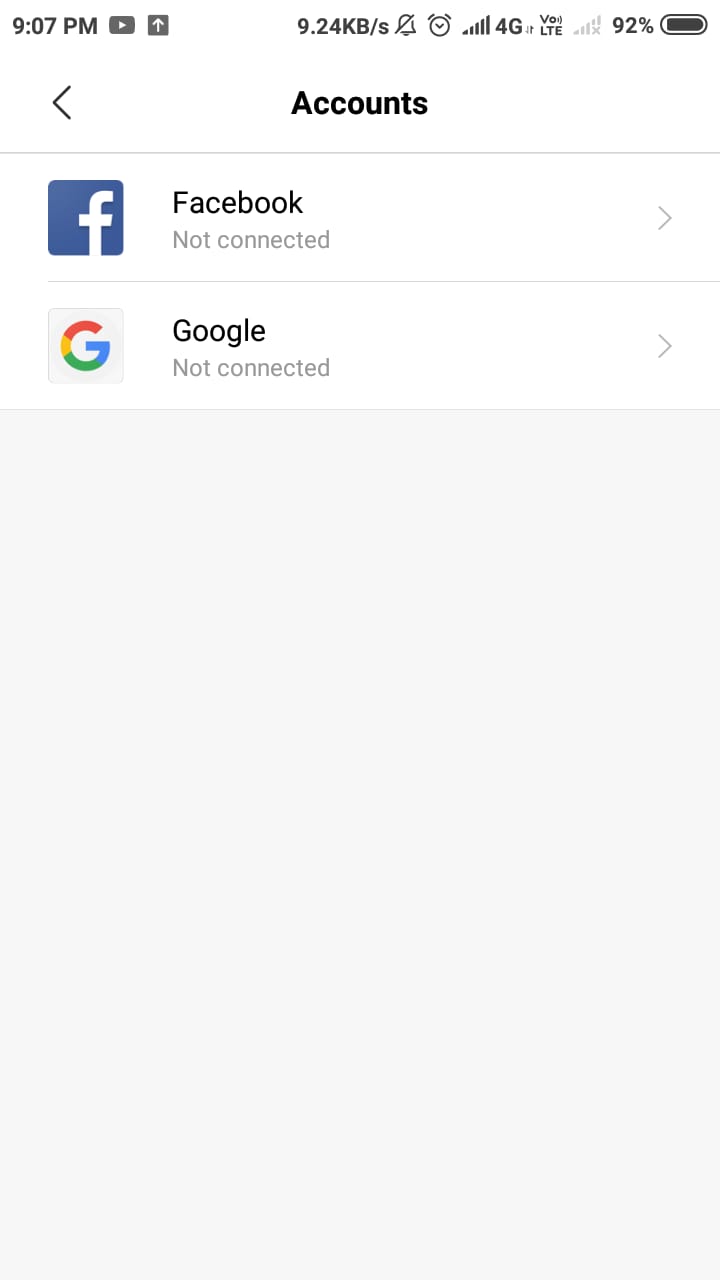The screenshot depicts the account page of a mobile device, captured at precisely 9:07 PM, as indicated by the time displayed at the top left corner. The status bar is densely populated with various icons including the YouTube icon, indicators for download and upload speeds, a mute button, a full-strength network signal bar, an active alarm icon, and a voice over LTE (VoLTE) symbol. Additionally, there is an indication that the second SIM slot is unoccupied (SIM 2), and the device's battery level is critically low, sitting at just 2%. On the screen, the account settings are visible, showing that connections to both Facebook and Google accounts are not established.